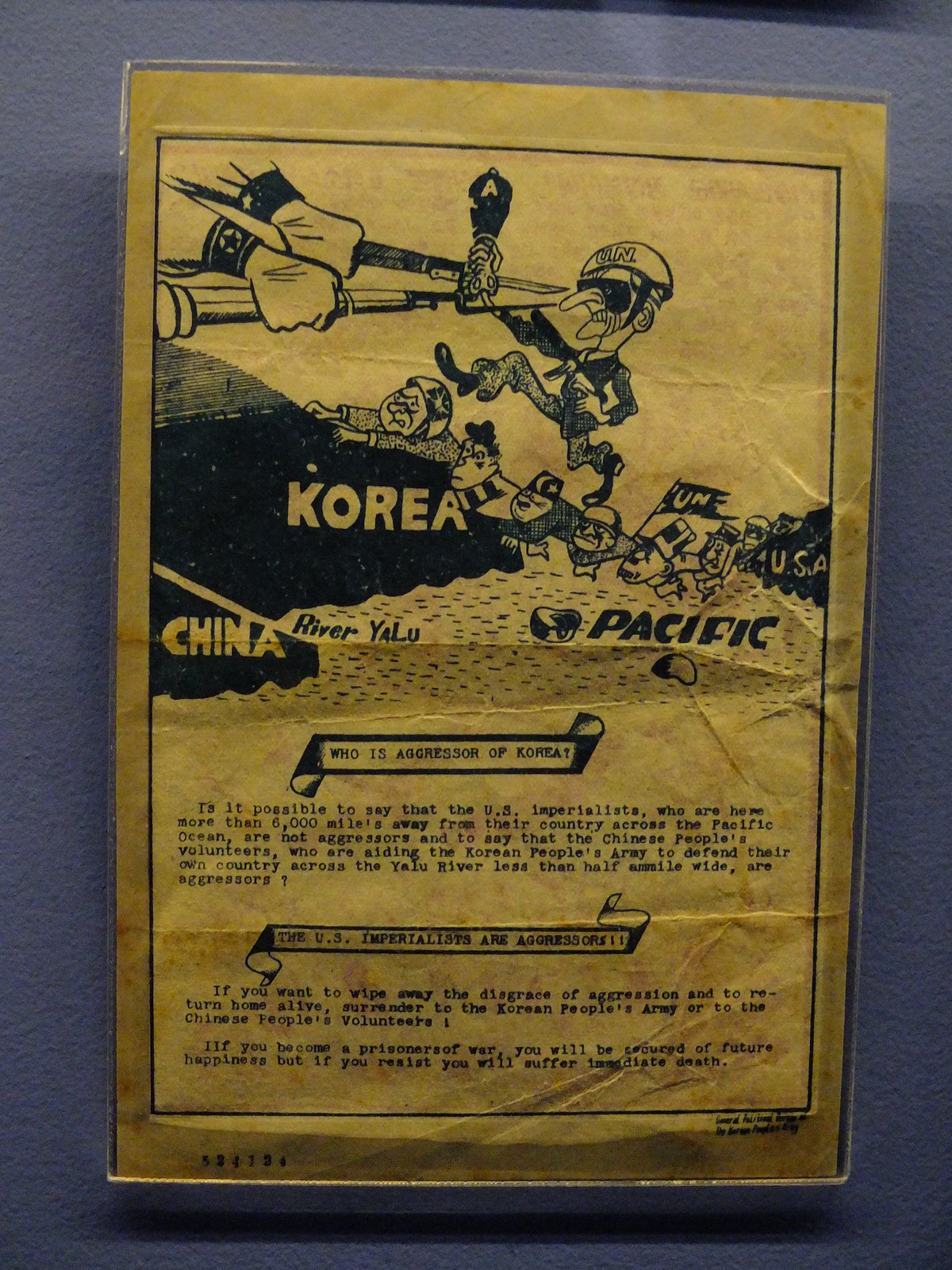This image features a single, detailed object centered against a purplish-blue backdrop. The main object is a worn, vintage poster or flyer, showcasing a political cartoon style. The paper of the poster is yellowed and wrinkled, indicating its age. At the top of the poster, the words "Korea," "China," "River Yalu," and "Pacific" are prominently displayed. The main illustration depicts a caricature of a soldier with a "UN" helmet, running towards two hands in the upper left corner holding a bayonet-equipped rifle. Beneath the running soldier, two figures lie on the ground—one marked with a "UN" flag. On the poster, text asks, "Who is the aggressor of Korea?" and criticizes U.S. imperialism. The overall color palette includes shades of purple, yellow, tan, black, and gray. This faded, brownish poster's text and imagery grimly recall the Korean War, showcasing a blend of aggressive and defensive symbols and highlighting the geopolitical tensions of the era.